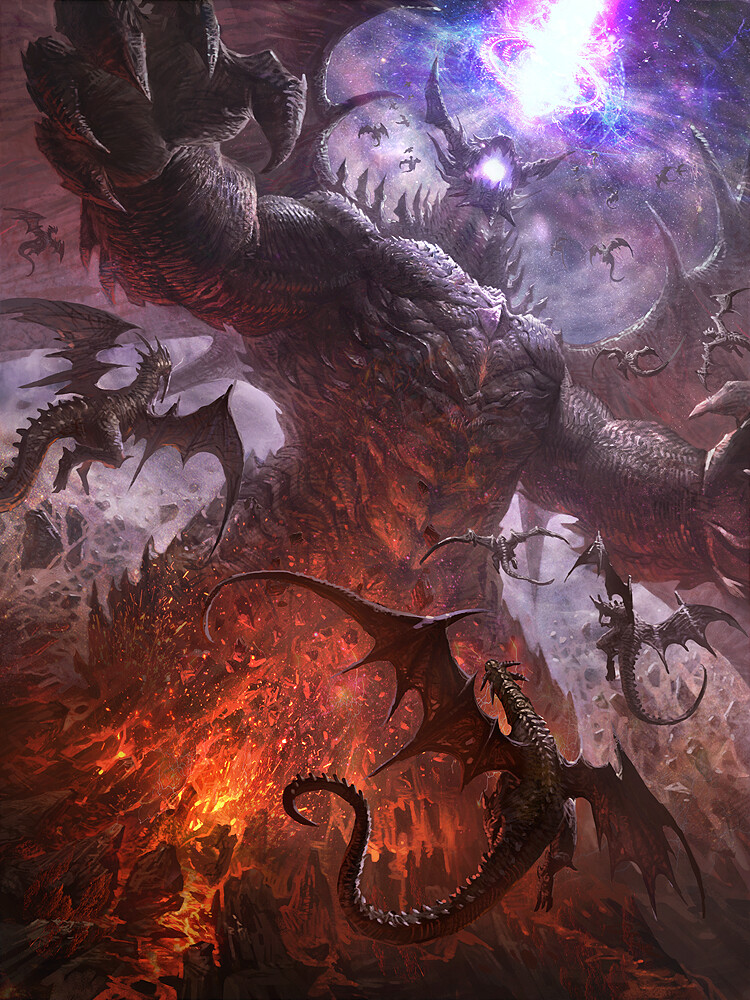This highly detailed digital fantasy artwork showcases a vertical portrait of a colossal, anthropomorphic dragon. The muscular beast stands on its hind legs, its massive chest and abdomen prominently displayed as it unleashes a deafening roar. Inside its gaping mouth, a vivid purple light glows ominously. The dragon’s powerful arms are outstretched, revealing its thick claws and sharp nails. Sharp spikes adorn its neck, giving it an even more menacing appearance. 

It appears to erupt from the earth, with jagged rocks exploding upwards around its feet, illuminated by a fiery red, lava-like glow. Surrounding the giant dragon are numerous smaller dragons, their elongated hooked wings and spiked tails adding to the chaotic scene. These smaller creatures are primarily gray in color, accentuating the dramatic atmosphere. 

The viewer's perspective looks up through the outstretched wings of the central dragon, revealing a vibrant blue sky filled with even more dragons in flight. Dominating the sky is a brilliant bolt of light emanating from what appears to be a black hole, casting an intense and ethereal glow over the entire scene.